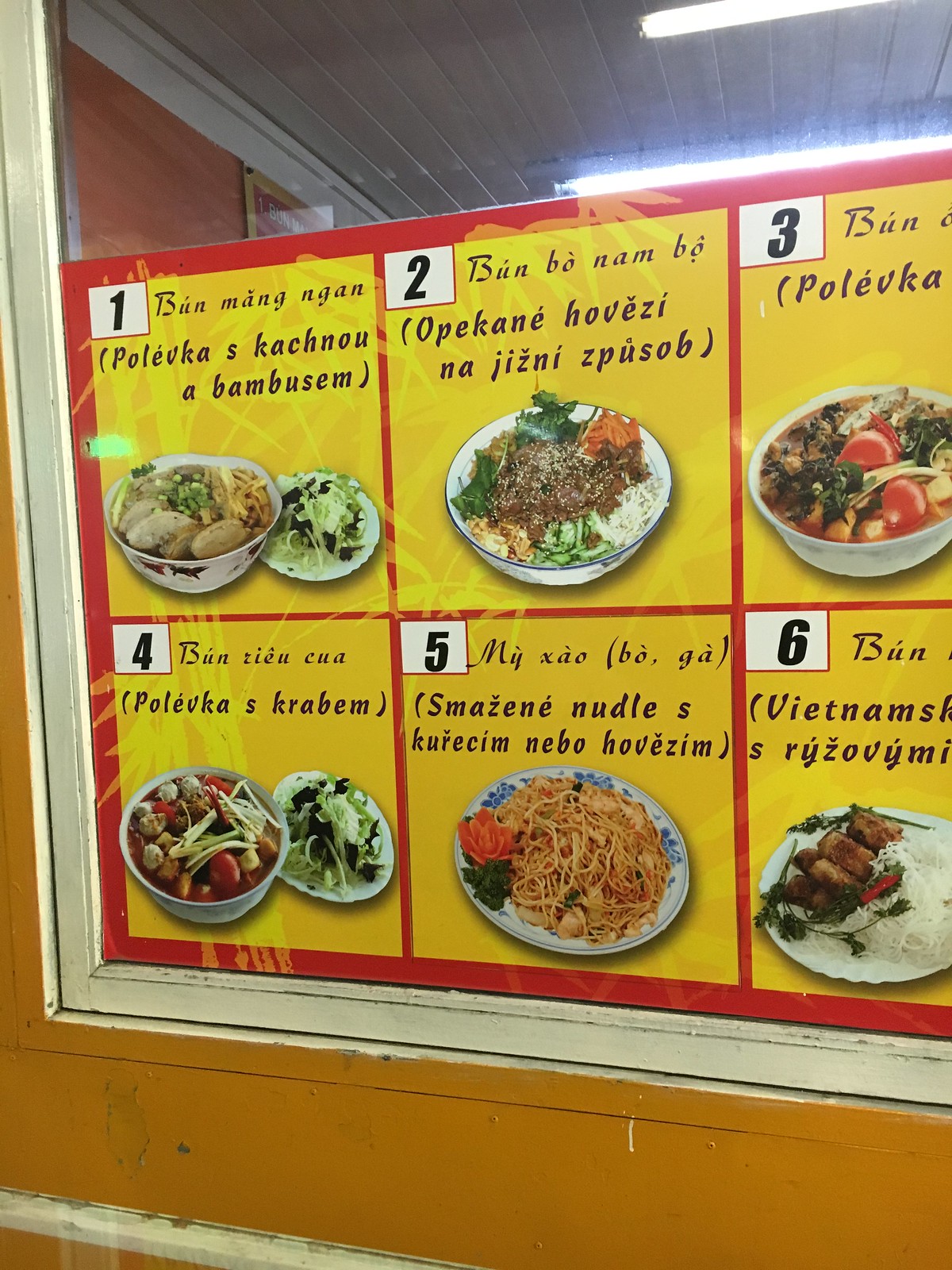A brightly colored orange building serves as the backdrop for this photograph, showcasing a large window adorned with a prominent menu placed to entice passersby. Positioned to grab the attention of those strolling down the street, the menu features vibrant images of various dishes, aiming to lure customers inside. The text on the menu is in an unidentified Asian language, suggesting the restaurant specializes in Asian cuisine, potentially Vietnamese.

The menu is organized into six options, numbered 1 through 6, with the first three choices displayed on the top row and the remaining three on the bottom row. Each item includes a picture and the name of the dish in prominent text. 

1. The first dish appears to be a type of soup, accompanied by a small plate of salad. Given the visual cues, this could be a type of pho, though it is labeled with different text, possibly indicating 'bun,' 'main,' 'don,' 'hula vega,' 'cashew,' or 'bamboo sum,' though these names are speculative.
   
2. The second dish resembles vermicelli noodles complemented by various trimmings and a portion of beef, reinforcing the notion that the cuisine is Vietnamese.

3. The third option presents another soup, distinct from pho, as it is garnished with large slices of tomato, indicating a unique flavor profile.

4. The fourth selection is also a soup, served with various accouterments like spiral-cut cucumber and lettuce, though the specific ingredients of the soup are unclear.

5. Dish number five is a classic stir-fry featuring noodles, offering a more familiar option to those who enjoy traditional noodle dishes.

6. The final option showcases pieces of chicken served alongside white vermicelli noodles, rounding out the menu with a hearty choice.

This detailed visual menu provides a glimpse into the rich variety of the restaurant's offerings, appealing to both the adventurous gourmet and those seeking the comforting flavors of authentic Vietnamese food.